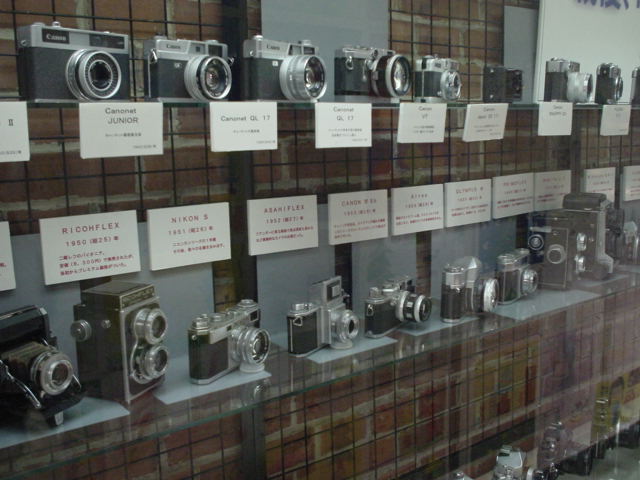The image depicts a detailed display of 20 vintage film cameras meticulously arranged on three shelves within a glass display case. The shelves, adorned with a red checkered pattern, contrast against the white walls, enhancing the retro aesthetic. Each camera is accompanied by a small placard detailing its model, brand, and year. The top shelf features approximately ten rectangular cameras, predominantly Canon models like the Canonet Junior, all with black lenses and branded text. The middle shelf offers a variety of black and silver-lensed cameras in different sizes, suggesting a collection of rare and desirable pieces, including the Rikom Flex from the 1950s with bilingual labeling in English and Chinese. Slightly visible at the bottom shelf are three additional cameras, hinting at an extensive collection, possibly indicating a museum or specialized camera store setting.